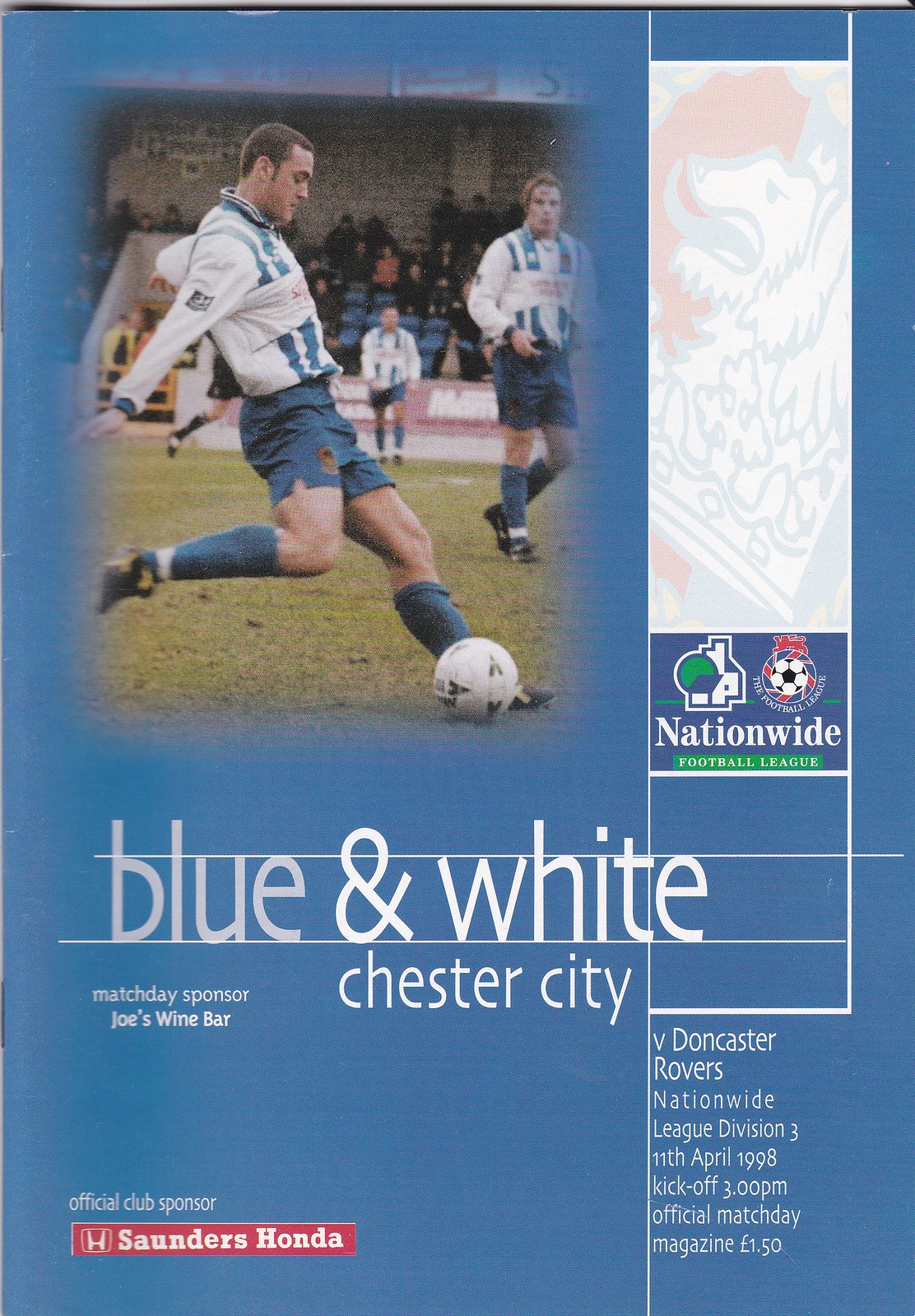The image is an advertisement for a soccer team set against a light blue background. In the upper left, there's a dynamic picture of a soccer player in action, with his leg kicked back and the ball in front of him. He is wearing a blue and white jersey paired with blue shorts. Surrounding him are several teammates, all in similar blue and white outfits. 

On the right-hand side, a banner prominently displays a close-up of the team's crest. Below this banner, the text reads "Nationwide Football League." Centrally located below the player’s picture, the words "Blue and White" are displayed, followed by "Chester City" beneath it. To the left of this, it indicates "Match Day Sponsor: Joe's Wine Bar." 

In the lower left corner, it says "Official Club Sponsor," with a red banner underneath that reads "Saunders Honda" in white letters, accompanied by the Honda logo. The lower right corner highlights that the team is playing against "Doncaster Rovers," specifying it is a "Nationwide League, Division 3" match scheduled for the "11th of April, 1998," with kickoff at "3 p.m." Finally, it is noted that this is the "Official Match Day Magazine" along with the price.